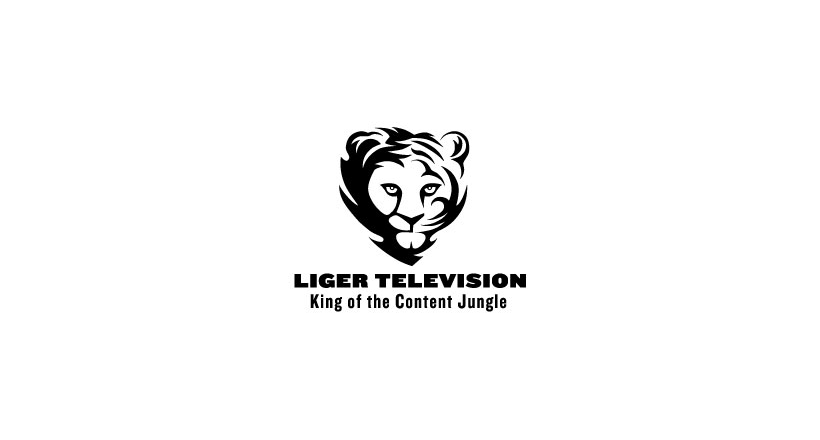The image is a black and white logo set against a white background. The logo features the face of a liger, which is a cross between a lion and a tiger. The liger's face, detailed with distinct stripes and a neutral yet somewhat defiant expression, is the central element. Above the head, the text reads in bold uppercase letters, "LIGER TELEVISION." Directly below this, in smaller, mixed-case text, is the slogan "King of the Content Jungle," with only the initial letters of "King," "Content," and "Jungle" capitalized. The entire logo, including the text and image, has a minimalistic design, making it appear as a small, yet striking, icon.